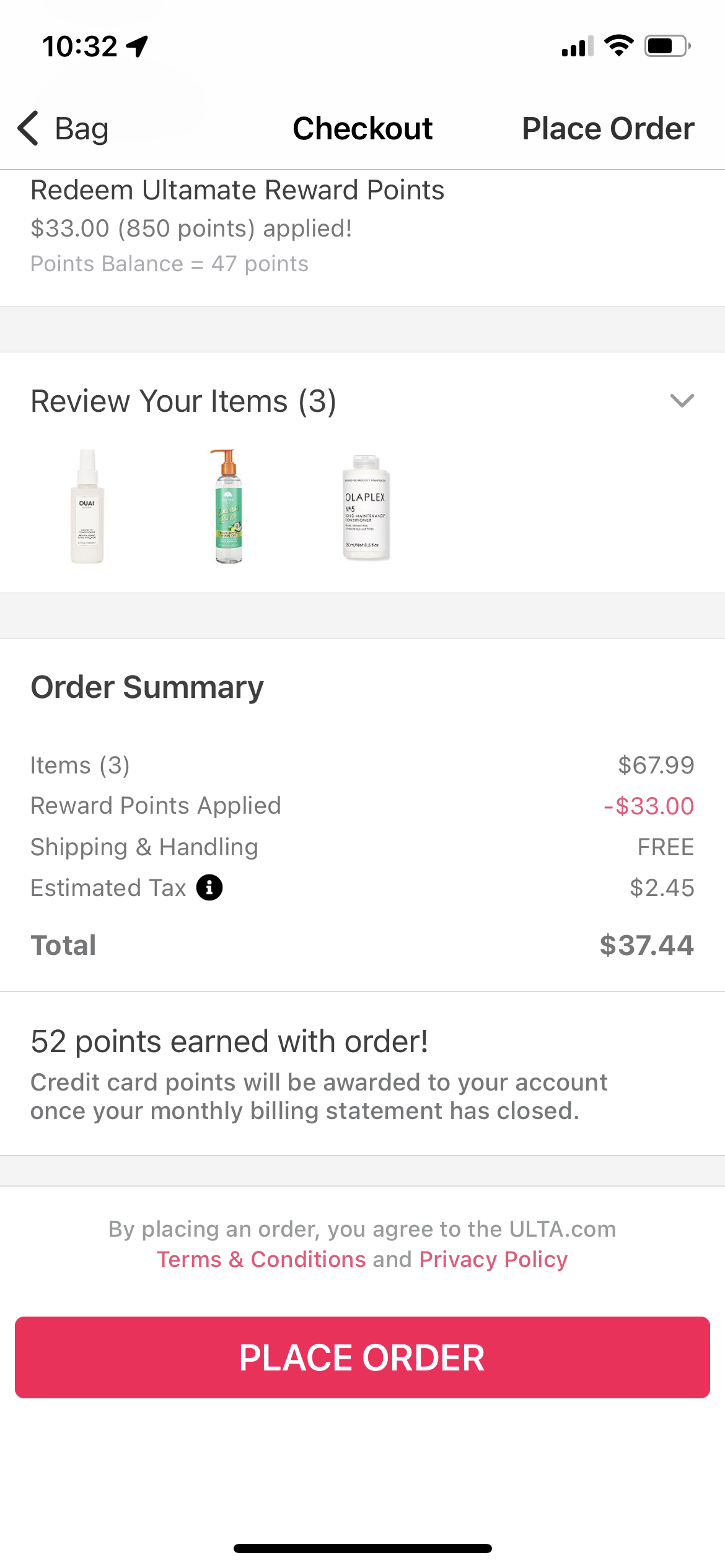The screenshot shows a detailed checkout summary on the Ulta.com website. The top-left corner displays the time, 10:32, while the top-right corner features standard mobile icons for signal strength, Wi-Fi, and battery status. The main section of the screen includes several buttons labeled "Bag", "Checkout", "Place Order", and "Redeem Ultimate Reward Points." Below, it indicates that $33 has been redeemed from 850 points, with a remaining points balance of 47 points.

The review section highlights three bottles as the items to be purchased. The order summary lists the total item cost as $367.99, with $33 deducted due to applied reward points, resulting in free shipping and handling. The tax is calculated at $245, leading to a final total of $37.44. The order will earn 52 points, and it's noted that additional credit card points will be awarded at the end of the monthly billing cycle. The screen concludes with a statement that placing the order signifies agreement to Ulta.com's terms and conditions and privacy policy, with a "Place Order" button situated above a black dividing line.